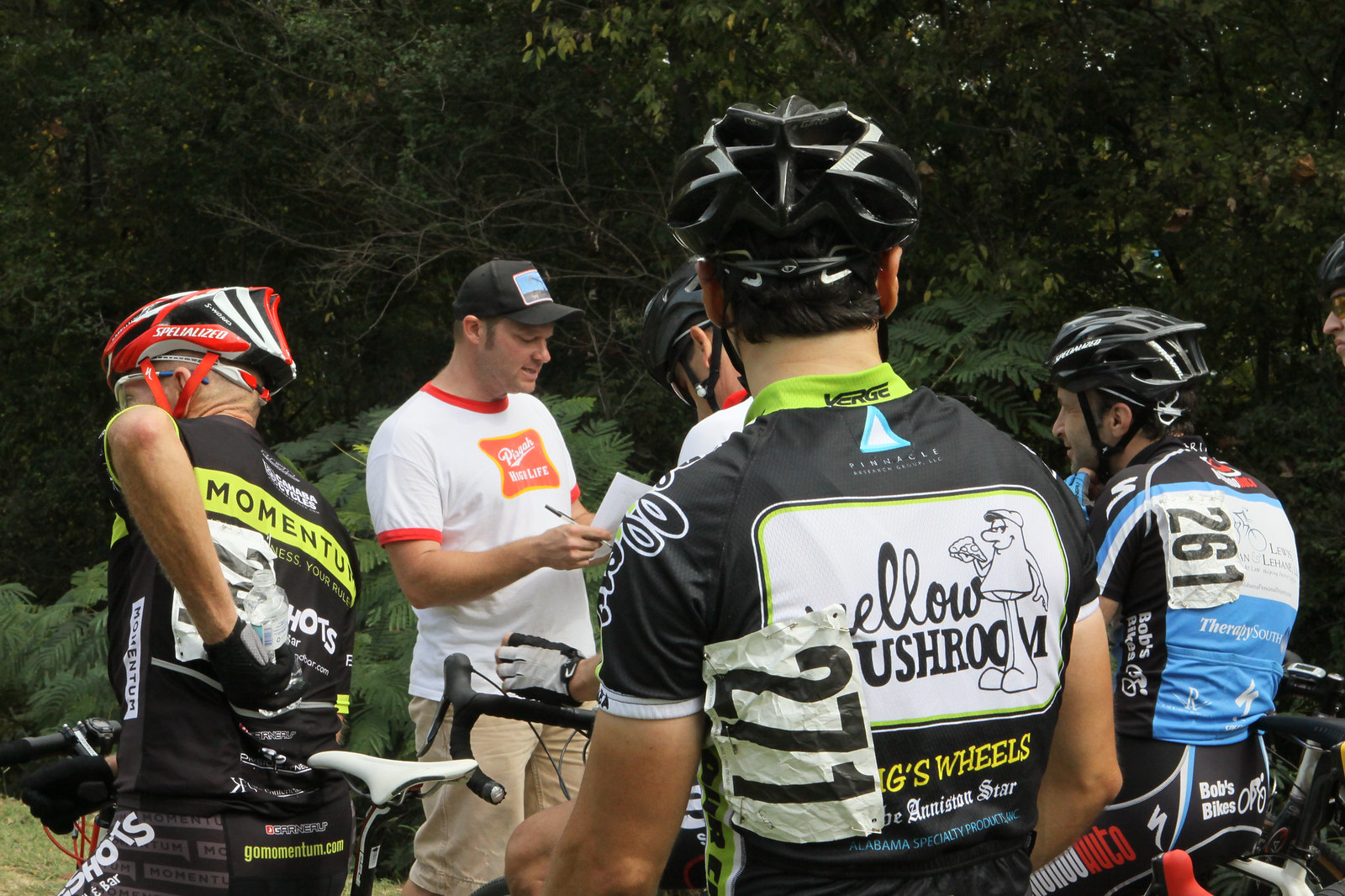In this horizontal rectangular image, a group of men is preparing for a bicycle race, staged against a backdrop of ferns and trees. The scene captures five individuals, four of whom are cyclists dressed in tight-fitting, logo-adorned racing gear, each with numbers on their backs for identification: number 271 on the man in the foreground, 261 on the man to his right, and the numbers on the other cyclists are less visible due to their positioning. The cyclists wear black helmets with visors, while their colorful jerseys feature combinations of neon yellow, black, white, and blue. On the far left, a man wearing a neon yellow and black jersey is partially visible, showing the seat of his bicycle. To the right, a cyclist in a black and blue jersey is only visible from the back. 

A significant figure in the scene is a man in a Miller High Life shirt, white with red seams and black text, who appears to be a race official. He stands holding a piece of paper and a pencil, likely giving instructions or checking in the participants. His outfit is completed with a black hat and khaki shorts. All the participants, including the race official, are wearing helmets, emphasizing the race's safety protocols. The mood suggests a moment just before the start of the race, with the cyclists gearing up and the official ensuring everything is in order.